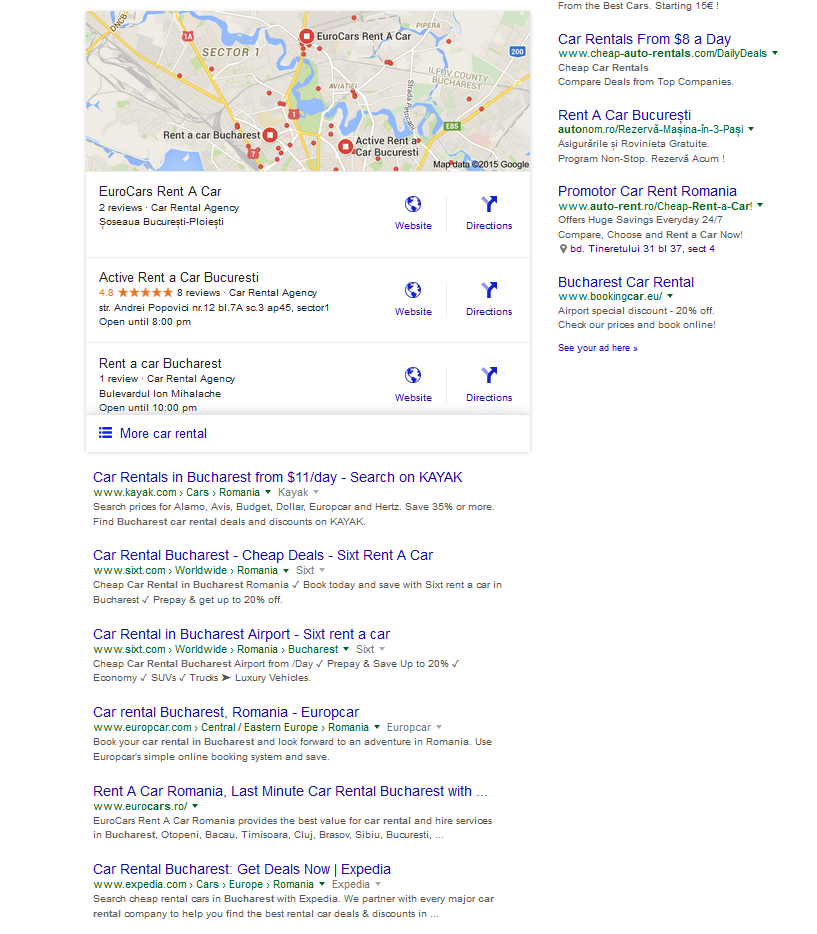The image depicts a Google search results page for car rental agencies in Bucharest. At the top of the page, a detailed map is featured, displaying multiple red location markers. These markers represent various car rental services across the city. Prominent locations mentioned on the map include Sector One and other areas in Bucharest.

Below the map, the first listing is for "Eurocars," identified as a car rental agency with two reviews. The listing provides a website link and directions, situated in a location with an unpronounceable name. The next listing features "Active Rent-a-Car Bucharesti," boasting a high rating of 4.8 stars based on eight reviews, also categorized as a car rental agency. Another notable listing is "Rent-a-Car Bucharest."

The search results further showcase advertisements and additional links for car rental services. The first advertisement highlights car rentals in Bucharest starting from $11 per day available on Kayak.com. Subsequent links promote car rental deals from companies like Sixt Rent-a-Car, with mentions of their services at Bucharest Airport. Other notable websites include Europcar.com, Eurocars.ro, and Expedia.

Adjacent to the map on the right-hand side, there are more condensed listings of similar car rental agencies, offering quick access to their respective services.